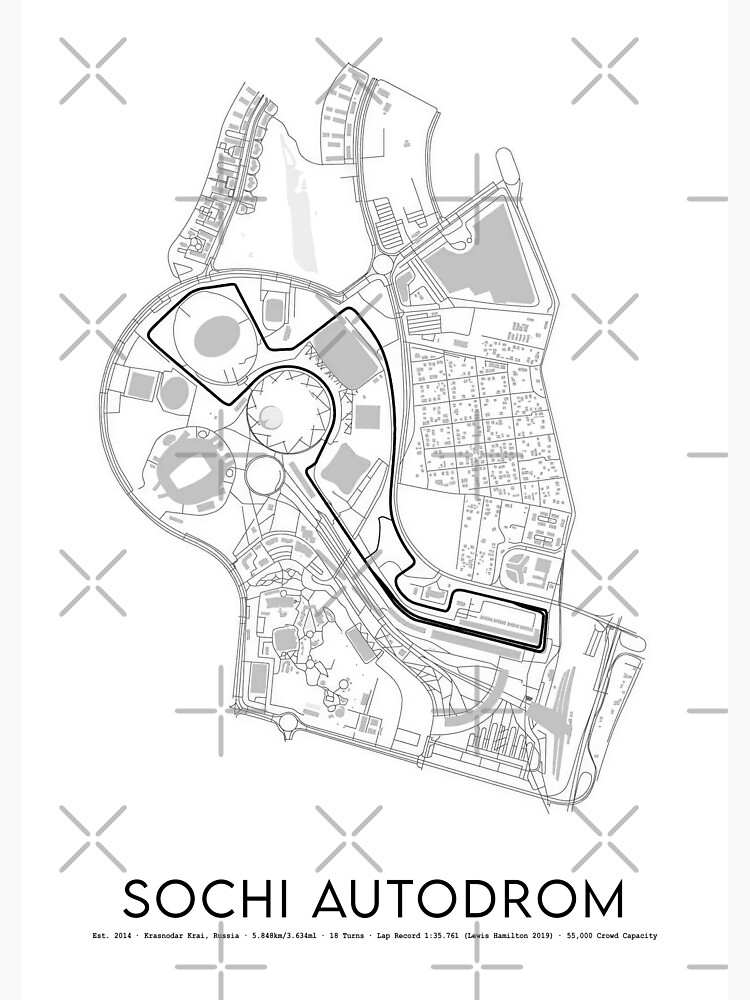This black-and-white blueprint drawing is a detailed architectural sketch of the Sochi Autodrom, a racetrack located in Krasnodar Krai, Russia, and established in 2014. The image is viewed from the top down, presenting a schematic map marked with fine grey lines depicting pathways, streets, and various sectors. Prominently featured is a dark line that highlights the 5.848-kilometer (3.634 miles) track with 18 challenging turns. A specific portion of the map is accentuated with a darker black outline, possibly indicating significant sections of the track or facility. Notably, the bottom of the image displays large black text reading "Sochi Autodrom," along with finer print detailing its notable features such as a crowd capacity of 55,000 and the lap record of 1:35.761 set by Lewis Hamilton in 2019.